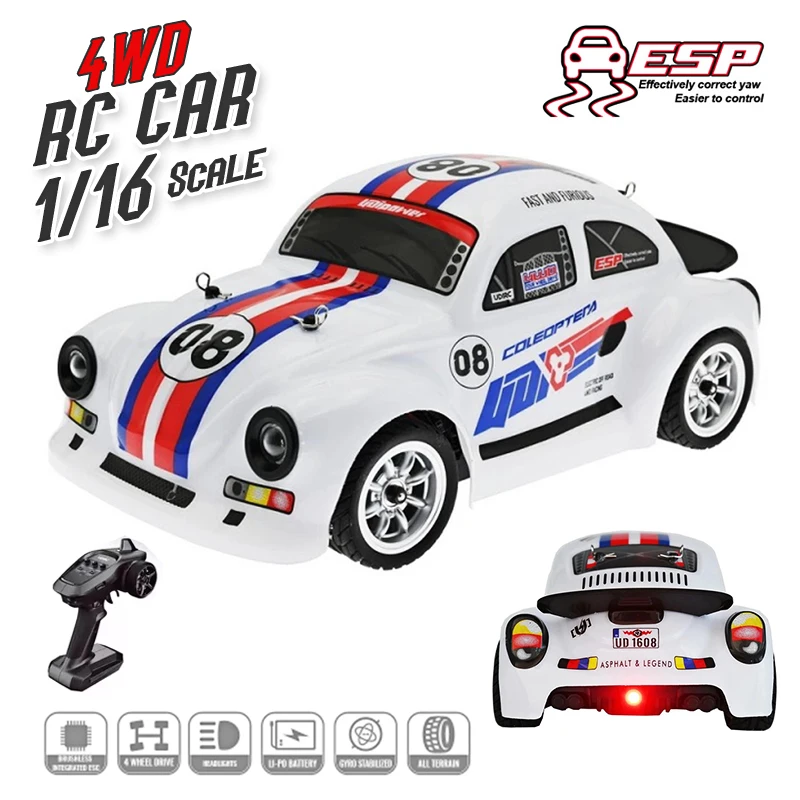This image is a detailed advertisement for a 1/16th scale, four-wheel-drive, remote control car modeled after a white Volkswagen Beetle race car. It features distinctive red, white, and blue racing stripes running from the hood, over the roof, and down to the rear. Prominently displayed on the hood within a white circle is the racing number 08. The car's driver's side door bears a blue, red, and white logo. The headlights are designed to resemble eyeballs, adding a playful touch to its appearance. 

The advertisement highlights several features: it mentions "ESP, effectively correct Y-A-W, easier to control" in the top right corner, suggesting enhanced maneuverability. The top left corner declares "Four Wheel Drive RC Car 1/16th Scale." The bottom left corner features an image of the remote control, while the bottom right shows the back of the car, equipped with a license plate reading "Asphalt and Legend," and a black fin. At the bottom of the ad, six gray icons detail additional features, including four-wheel drive, functional headlights, a battery indicator, and all-terrain capability, among others.